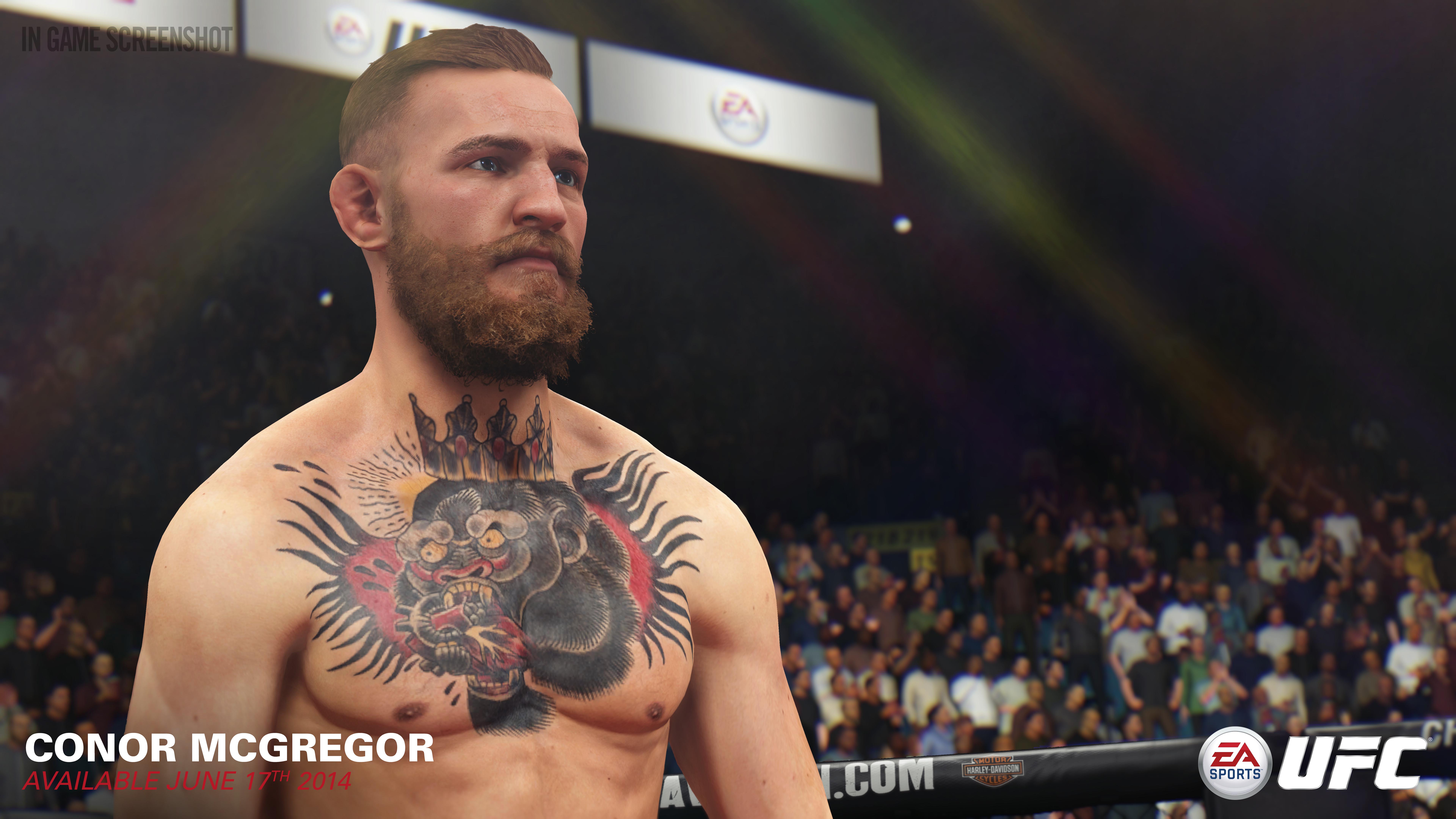In this detailed image, we see the UFC fighter Conor McGregor standing shirtless against a dark, indoor background filled with a massive crowd of people. Illuminated by diagonal beams of yellow and red light on the left and right, the scene is vibrant and intense. Above the crowd, three signs hang from the ceiling; one prominently features the UFC logo, while another displays the EA Sports logo in a white circle with red and blue text in the top left and bottom right corners. 

Conor McGregor, positioned on the left, has a distinctive reddish-brown beard and sleeked-back hair. His muscular chest and shoulder area are adorned with a dramatic tattoo, depicting what appears to be a black crowned beast extending up to his neck with elements of red and yellow in the design. His stern expression adds to the intense atmosphere of the scene. 

In white text at the bottom left, it reads "Conor McGregor," and just below that, in red text, it states "Available June 17, 2014." At the top of the image, on the left, it notes "In-game screenshot," indicating that this is a digital rendering likely from a video game. The crowd fades into darkness as it ascends, making the lower tiers more visible than the upper ones, thus highlighting the density and excitement of the audience.